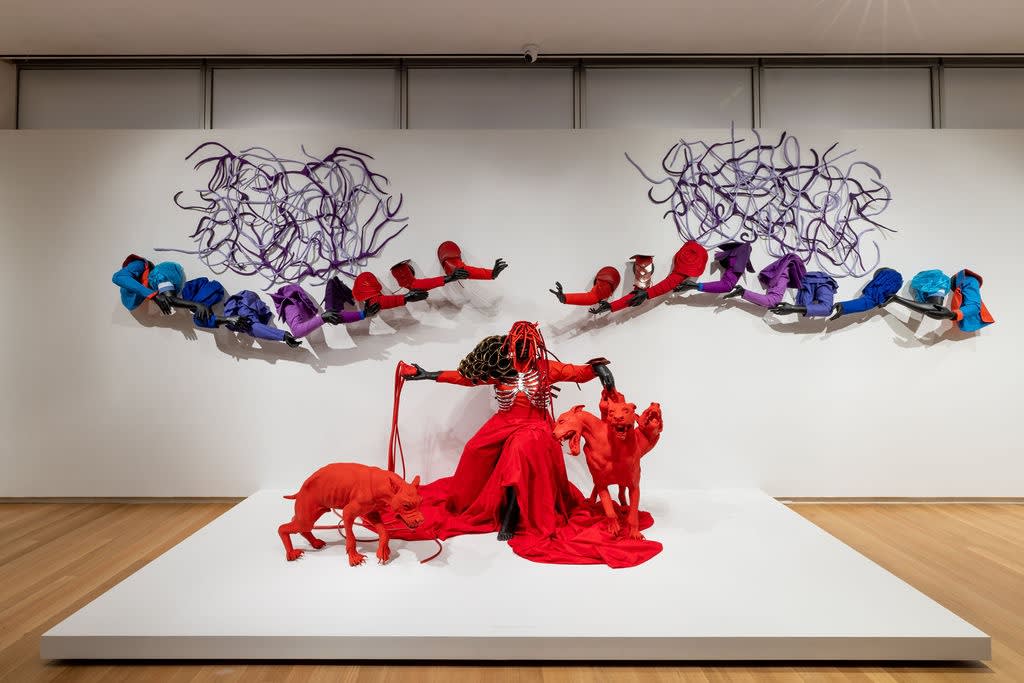The image captures a captivating art installation in a museum gallery. The central figure in this installation is a striking red character with white ribs exposed, adorned in a gothic red dress and possessing black hands, feet, and an indistinct black face. This eerie figure is seated on a white platform and holds two leashes: one attached to a menacing, three-headed demon-like dog on the left, and the other connected to a single-headed red dog on the right. The background features a white wall with multicolored, bent arms jutting out—left arms on the right side and right arms on the left side—each clad in sleeves transitioning from blue to purple to red. These arms add to the surreal and somewhat kitschy atmosphere of the installation. The gallery’s floor is of polished hardwood, providing a contrasting warm tone to the otherwise startling display. Purple string-like scribbles adorn the wall above the arms, further enhancing the composition's abstract and unsettling nature.